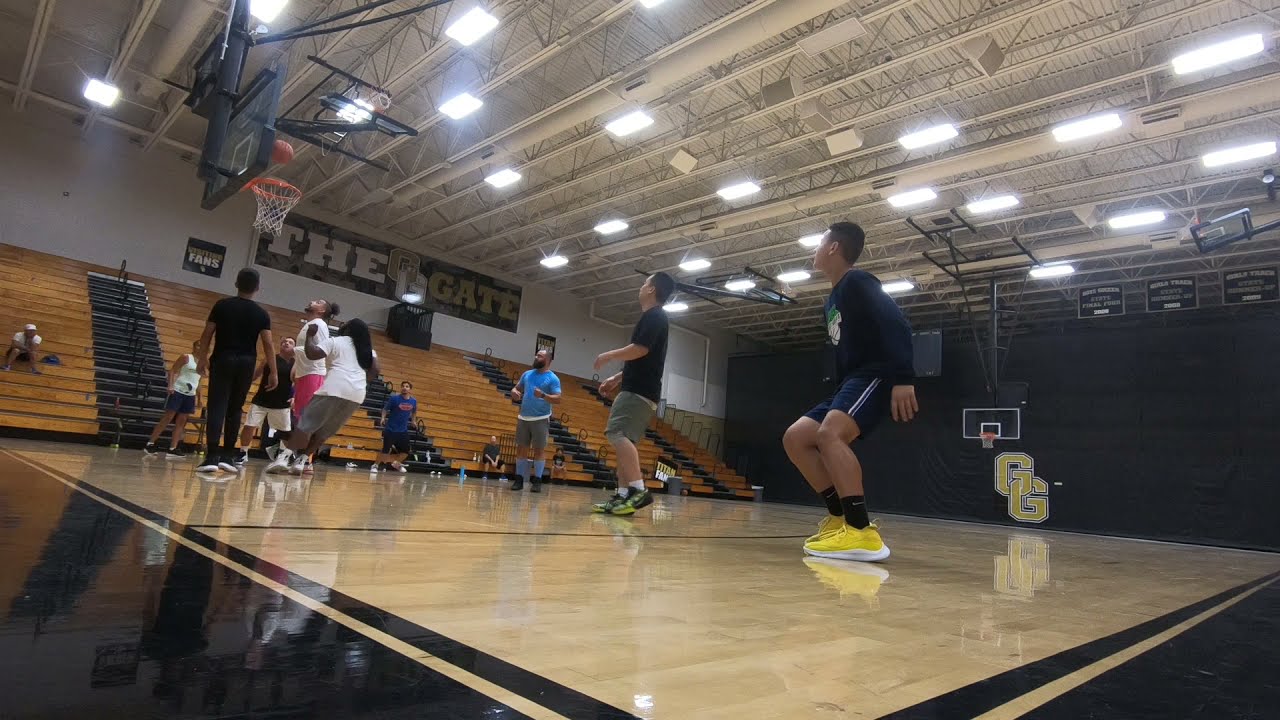This photograph captures an indoor gymnasium centered on a casual basketball game. At the forefront, slightly to the right, stands a boy in distinct yellow and white shoes paired with black socks, blue and white shorts with white stripes, and a blue jacket or hoodie featuring an insignia on the front. Nearby, to his left, is another boy clad in a black and gray shirt and shorts. To his other side stands an older man in a blue shirt and gray shorts. Further left, a group of students, wearing various colored shirts and pants, are gathered attentively, watching a basketball hovering just above the hoop, poised to fall through. The gymnasium floor shines brightly with a black and beige wood design bordered by a black stripe. In the background, a few spectators are seated on the bleachers. Dominating the scene above them, a large black and white banner prominently displays the words "The Gate," with an insignia of two interlocking Gs. The captured moment shows a total of seven or eight players on the court, each with their gaze fixed on the ball above the basket, poised in anticipation of its descent.